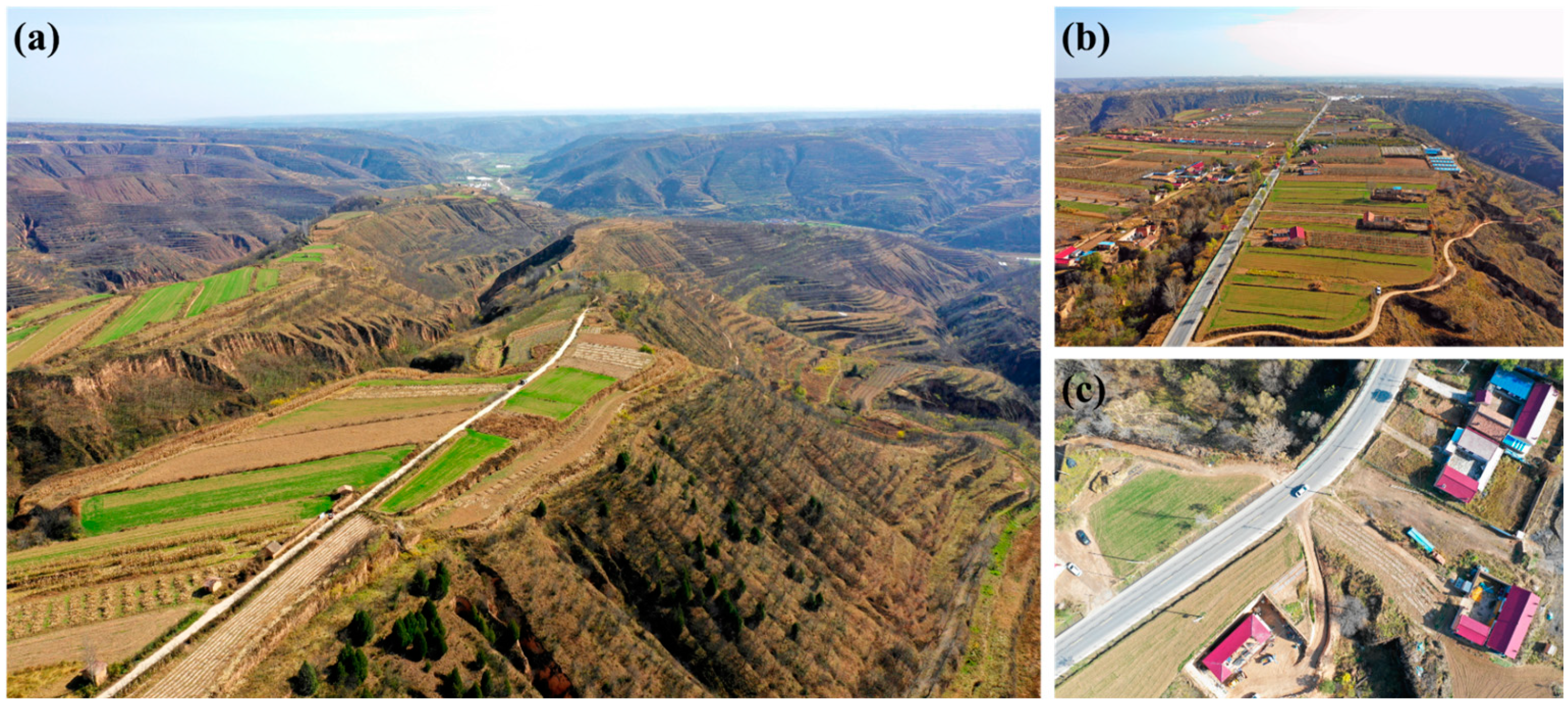This is a photographic outdoor triptych of aerial views labeled A, B, and C, positioned left to right. The largest image, A, showcases a dramatic overhead shot of a long, white road—or possibly a railroad—running through a green and brown embankment atop a cliff. The scene includes rocky inclines leading to a level plateau, visible green fields, distant mountains, and a clear blue sky. Image B presents a similarly steep and rugged terrain, featuring a straight highway that splits the land from bottom to top, with a winding road along a hill to the right and some buildings on the left. Image C zooms in closer on a rural landscape, highlighting a meandering gray road adjacent to a green field dotted with houses sporting red and blue roofs. The series collectively captures varying perspectives of lush farmlands, rolling hills, and mountainous regions, all basked in daylight.